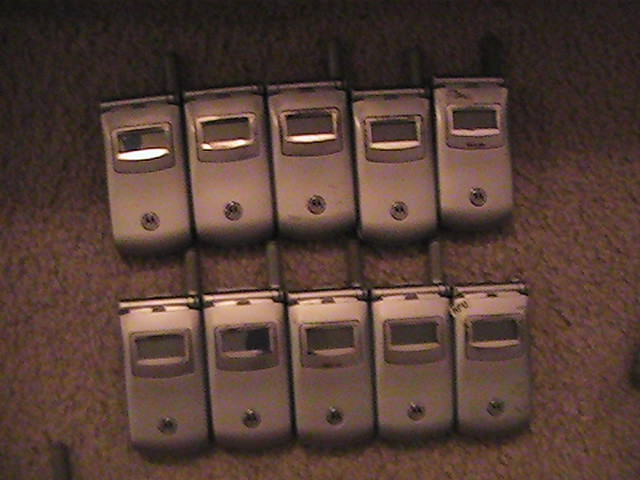The image is a dark, poor-quality color photo featuring ten silver flip-top cell phones, likely Motorola brand given the 'M' logo visible on them. The phones are arranged in two slightly uneven rows of five against a brown, possibly worn or dirty fabric background. Each phone has a small screen and a circular button with an 'M' logo at the bottom. Most phones possess a black antenna, although a few are missing this feature: namely, the second phone in the top row and the fifth phone in the bottom row. Despite the fuzzy autofocus, the silver detailing around the screens and antennas is noticeable.